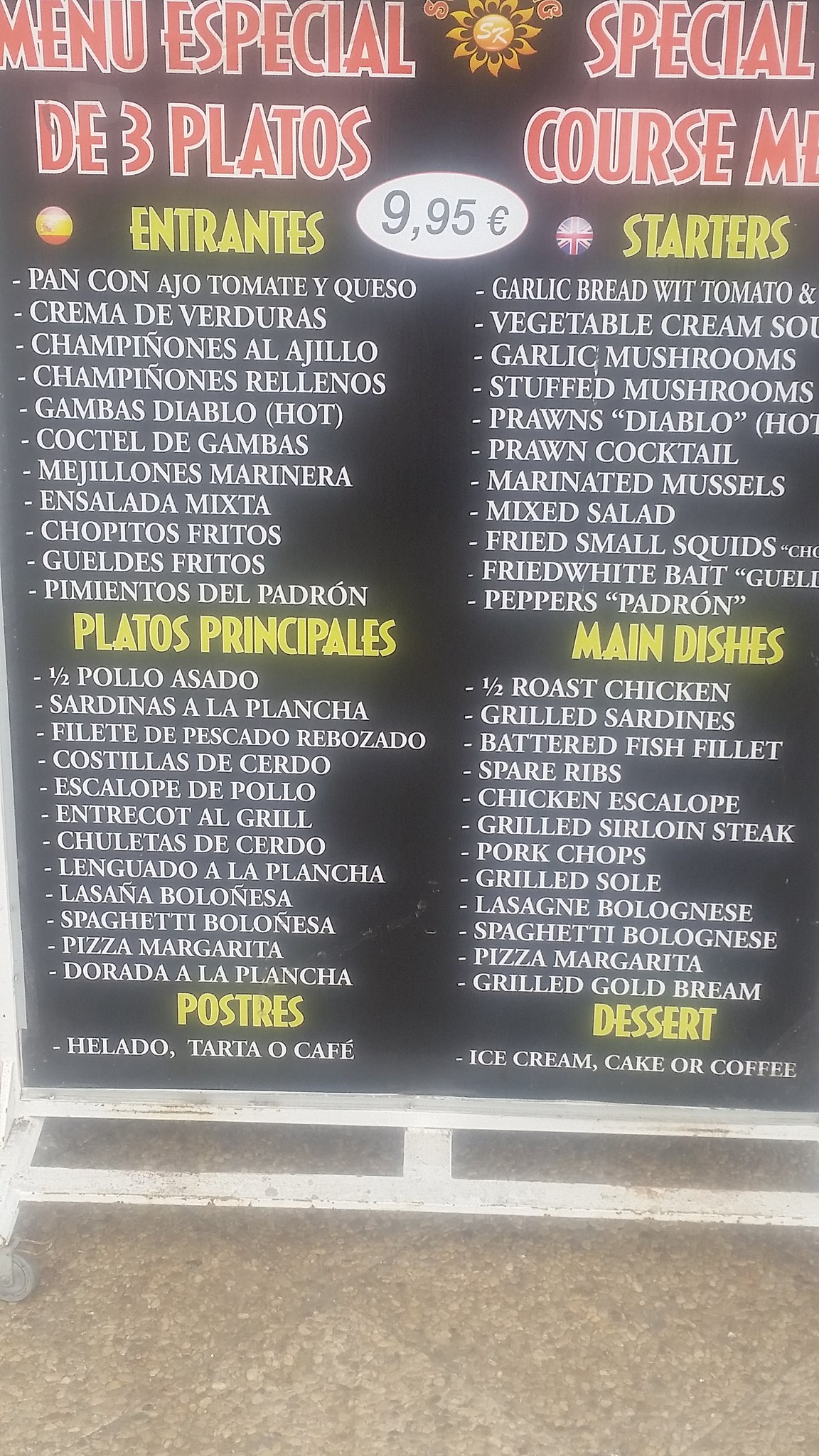This image features a European menu showcasing a special offer under the heading "Menu Especial de 3 Platos," which translates to "Special 3-Course Menu." Priced at €9.95, the menu presents a comprehensive selection for each course, highlighting the diversity of culinary delights.

The first section is titled "Entrantes" (Starters), listing items such as "Pan con Ajo" (Garlic Bread), "Tomates" (Tomatoes), "Queso" (Cheese), and "Crema de Verduras" (Vegetable Cream Soup). Each starter is designed to tantalize the taste buds, setting the stage for the main course.

The next section, "Platos Principales" (Main Courses), offers a variety of generously portioned dishes. Options include "Pollo Asado" (Grilled Chicken), "Spaghetti Bolognese" (Spaghetti with Meat Sauce), and "Pizza Margarita" (Margherita Pizza). These main dishes are crafted to cater to diverse palates and provide a hearty meal.

Finally, the "Postres" (Desserts) section tempts diners with sweet endings such as "Helado" (Ice Cream) and "Milkshake." These desserts add a delightful conclusion to the dining experience.

The menu titles are prominently highlighted in blue and yellow, ensuring easy navigation through the offerings. The universal price of €9.95 underscores the value proposition of this special menu, inviting patrons to enjoy a full three-course meal at an attractive price.